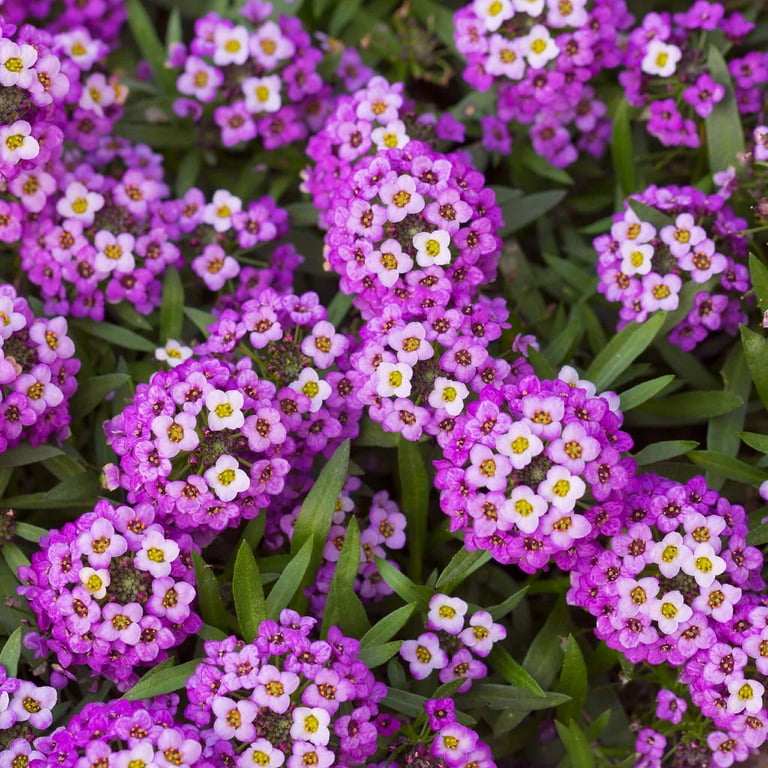This is an overhead, top-down aerial view of a vibrant field brimming with flowers. The image captures several clusters of flowers, each bundle appearing to be a composite flower made up of numerous smaller blooms. These clusters predominantly feature petals that transition from dark purple at the extremities to lighter purple and white towards their centers. Some flowers also exhibit a striking yellow-brown center. Scattered throughout the scene, thin green leaves with visible white veins peek out from beneath the floral clusters, adding to the lushness.

The arrangement forms a pattern; at the top of the image, there are approximately four bundles, each with purple petals transitioning to white and yellow centers. Along the sides, there are three similar bunches aligned vertically from top to bottom. In the center, the clusters fan out slightly, creating an almost inverted A-shape with one prominent cluster at the top. Across the middle of the image, three horizontally aligned clusters mirror the color pattern of purple edges and white centers. Lastly, the bottom left corner features another bundle that maintains this color scheme, lending a consistent and harmonious rhythm to the entire composition.